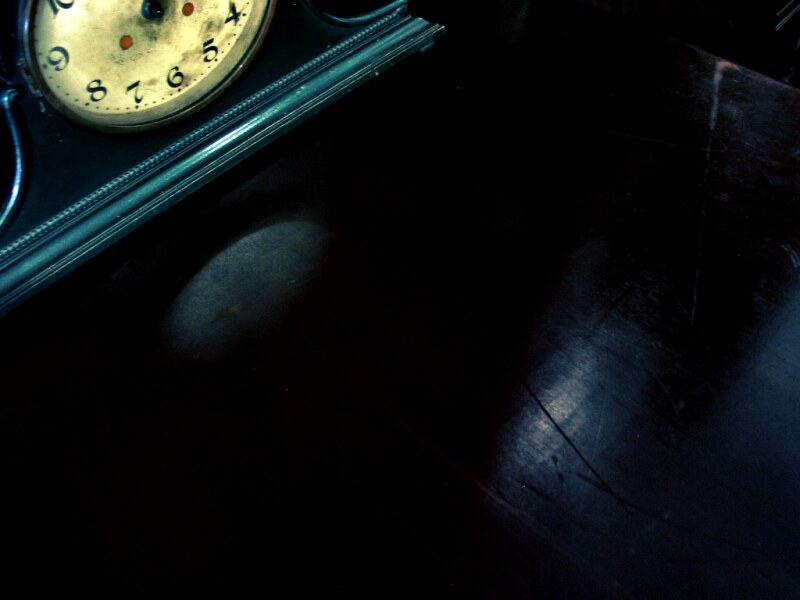The image presents a scene shrouded in darkness, lending a mysterious and somber tone. Dominating the top left corner is a partially visible, circular clock. The clock's face is predominantly a light yellow but is marred by dark stains, giving it a weathered look. Noteworthy are two small, red dots positioned near the center of the clock face, close to where the hands would intersect, although the hands themselves are obscured and seem to be pointing upward. The clock sits on a black, triangular ledge which appears to form its base. This ledge juts out into an arc-like opening beneath the clock, suggesting a sense of depth and layering in the composition. The base of the clock rests on a dark surface that resembles the corner of a table, marred with numerous scratches, underlining a sense of age and use. The pervasive darkness and subtle details create a hauntingly atmospheric image.